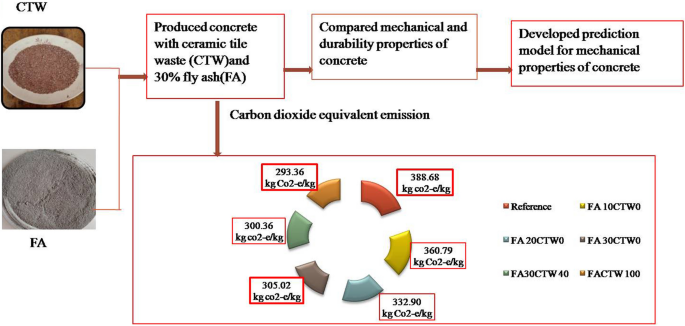This image is a detailed pictograph illustrating the carbon dioxide equivalent emissions associated with various concrete mixtures. At the top, there is a depiction of a plate containing a brownish substance labeled CTW (Ceramic Tile Waste) and, beneath it, another plate with a grayer substance. Both plates connect to a series of boxes with descriptive text. 

The first box is labeled "Produced concrete with ceramic tile waste (CTW) and 30% fly ash (FA)." An arrow points from this box to the next, which states "Compared mechanical and durability properties of concrete." Another arrow leads to a box that says "Developed prediction model for mechanical properties of concrete."

Below these boxes, a large circular chart features multiple colored segments, each representing different carbon dioxide equivalent emissions for various mixtures – these are labeled as follows: an orange segment at 293.36 kg CO2e, red at 388.68 kg, yellow at 360.79 kg, light blue at 332.90 kg, black at 305.02 kg, and light green at 300.36 kg. Each color corresponds to different mixes or reference values, providing a comparative visual of emissions data.

The overall layout effectively communicates the progressive steps of producing and analyzing concrete with ceramic tile waste and fly ash, culminating in the detailed portrayal of CO2 emissions with a color-coded pie chart indicating specific emission values.